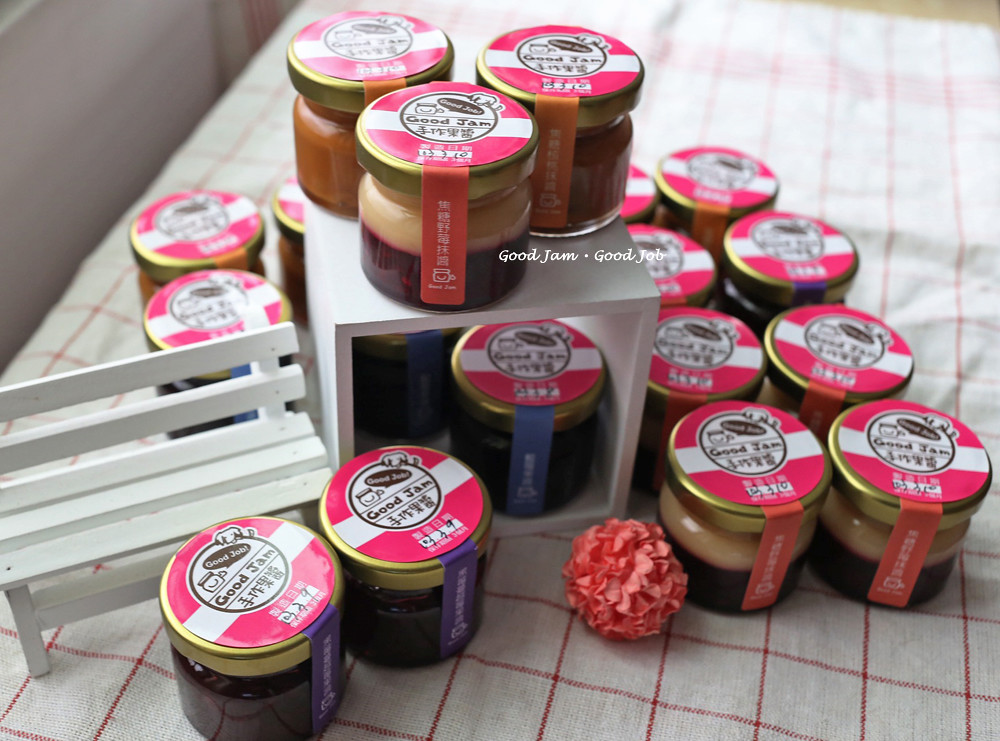The photograph showcases a well-arranged scene on a white tablecloth with small red lines forming large white checks. The main focus is a collection of 17 differing colorful jars of jam, meticulously displayed. Each jar's lid displays the phrase "good jam" followed by "good job" in a word bubble, both in English and accompanied by Japanese characters, indicating possible bilingual labeling. 

In the center, a small white open-ended box holds jam jars, with two jars inside and three neatly placed on top. To the left of this box stands a small toy replica of a white bench, with two jars positioned in front and two behind it, enhancing the playful yet orderly display. Also, near the box is a decorative touch - a pink flower ball, adding a subtle aesthetic element to the meticulously structured layout. The diverse jam colors range from vibrant reds to deep purples and rich oranges, indicating a variety of flavors within this visually appealing scene, likely intended as an engaging product photo for social media or a website.